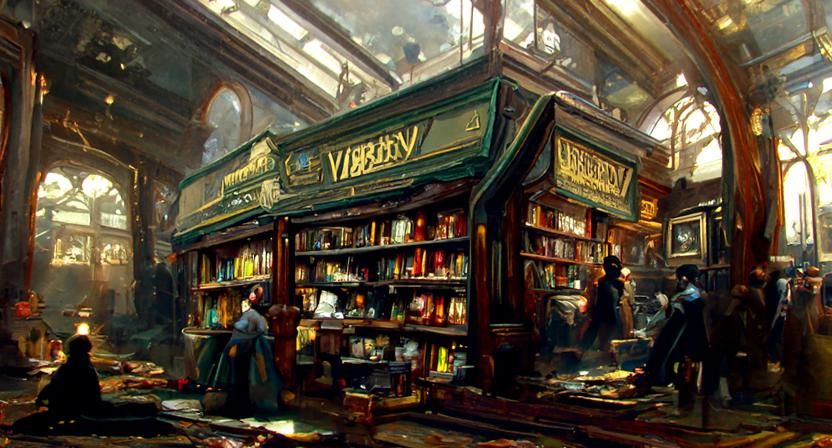The image depicts an interior scene within a grand building, likely a library or bookstore, featuring vivid elements that merge the real and the fantastic, suggesting it may be an AI-generated artwork or a detailed painting. The architecture includes tall arched walls on the right with large, bright windows that let in ample light, creating a serene ambiance. The ceiling is adorned with clear, vibrant glass panels that enhance the illumination below.

Central to the image is an expansive, multi-tiered bookshelf structure with deep, dark brown wooden shelves. The shelves are filled with a myriad of colorful books, with vibrant bookends in red, orange, and yellow hues. A striking feature is a green trim along the top of the shelving unit, adorned with golden writing that appears to name the establishment though it's not in English and somewhat ambiguous in its script.

There are three main sections of shelving: two long sides on the left and one shorter side on the right. People are scattered around the scene, browsing through the books. On the left, there is a mannequin in a blue dress amidst the shelves, while nearby, another person dressed in black appears to be a bookseller interacting with a buyer in a blue robe. The detailed observation of individuals engaging with the books adds life to the image, underscoring the atmosphere of a bustling yet old-world literary haven.